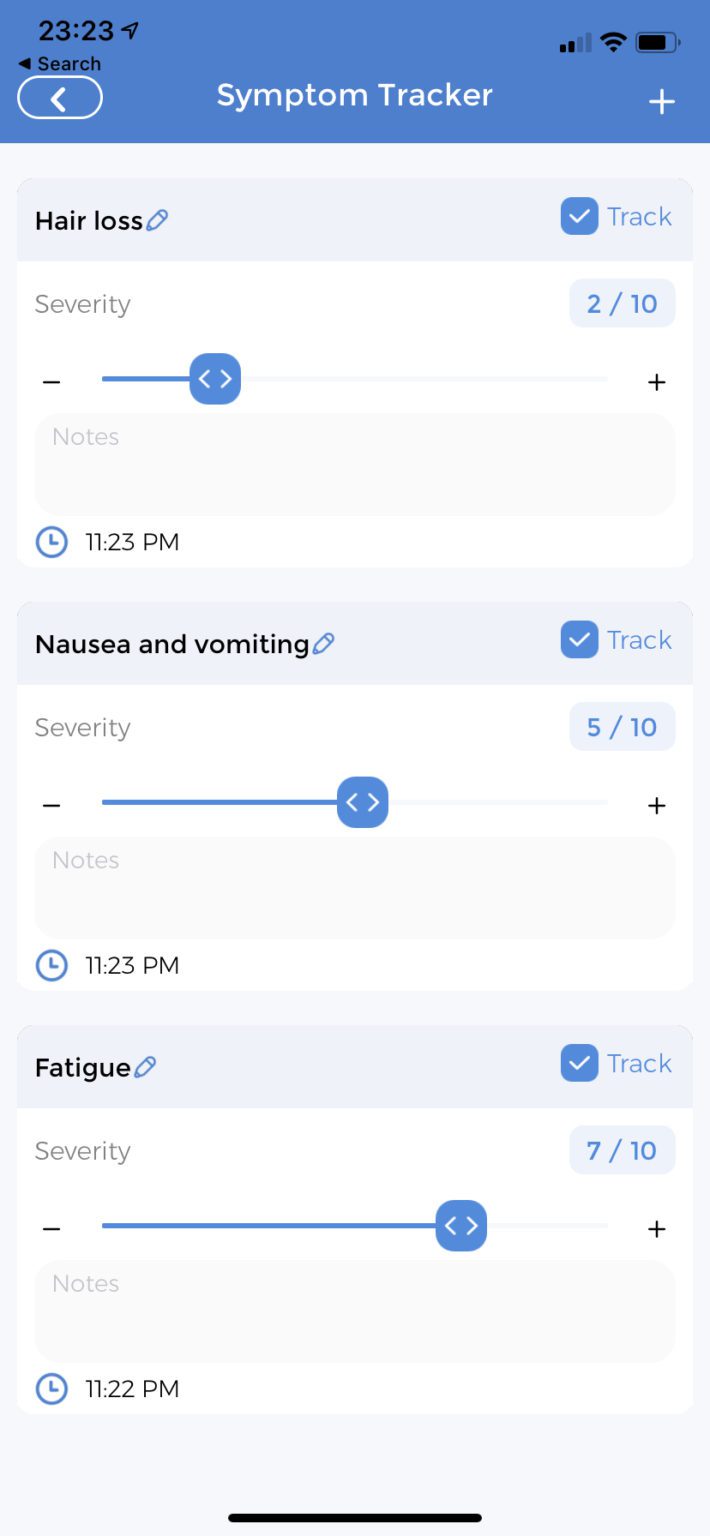This image appears to be a screenshot of a mobile app interface designed for tracking symptoms. At the top of the screen, the title "Symptom Tracker" is prominently displayed, accompanied by a back arrow on the left and a plus sign on the right, suggesting options to navigate back or add new entries.

The app interface is organized into several neatly labeled sections, each designed to facilitate easy symptom tracking. Each section features a gray header, and in the top right corner, there's a blue box with a checkmark labeled "Track," indicating active tracking for that symptom. A blue pencil icon on the left side of the header allows users to rename the symptom.

Within each section, users can see:
- **Symptom Name**: For example, "Hair Loss."
- **Severity**: Displayed as a number out of ten (e.g., 2/10).
- **Adjustable Slider**: Positioned beside plus (+) and minus (-) buttons to modify the severity level.
- **Notes Field**: For additional details or observations.
- **Timestamp**: Indicating the time of entry.

Three specific symptoms are listed in the screenshot:
1. **Hair Loss**: Tracked at 11:23 PM with a severity of 2/10.
2. **Nausea and Vomiting**: Also tracked at 11:23 PM, with a higher severity of 5/10.
3. **Fatigue**: Tracked at 11:22 PM, showing a severity of 7/10.

This symptom tracker app appears to be an effective tool for individuals managing health conditions, such as cancer, allowing them to monitor and document their symptoms in a streamlined and organized manner.